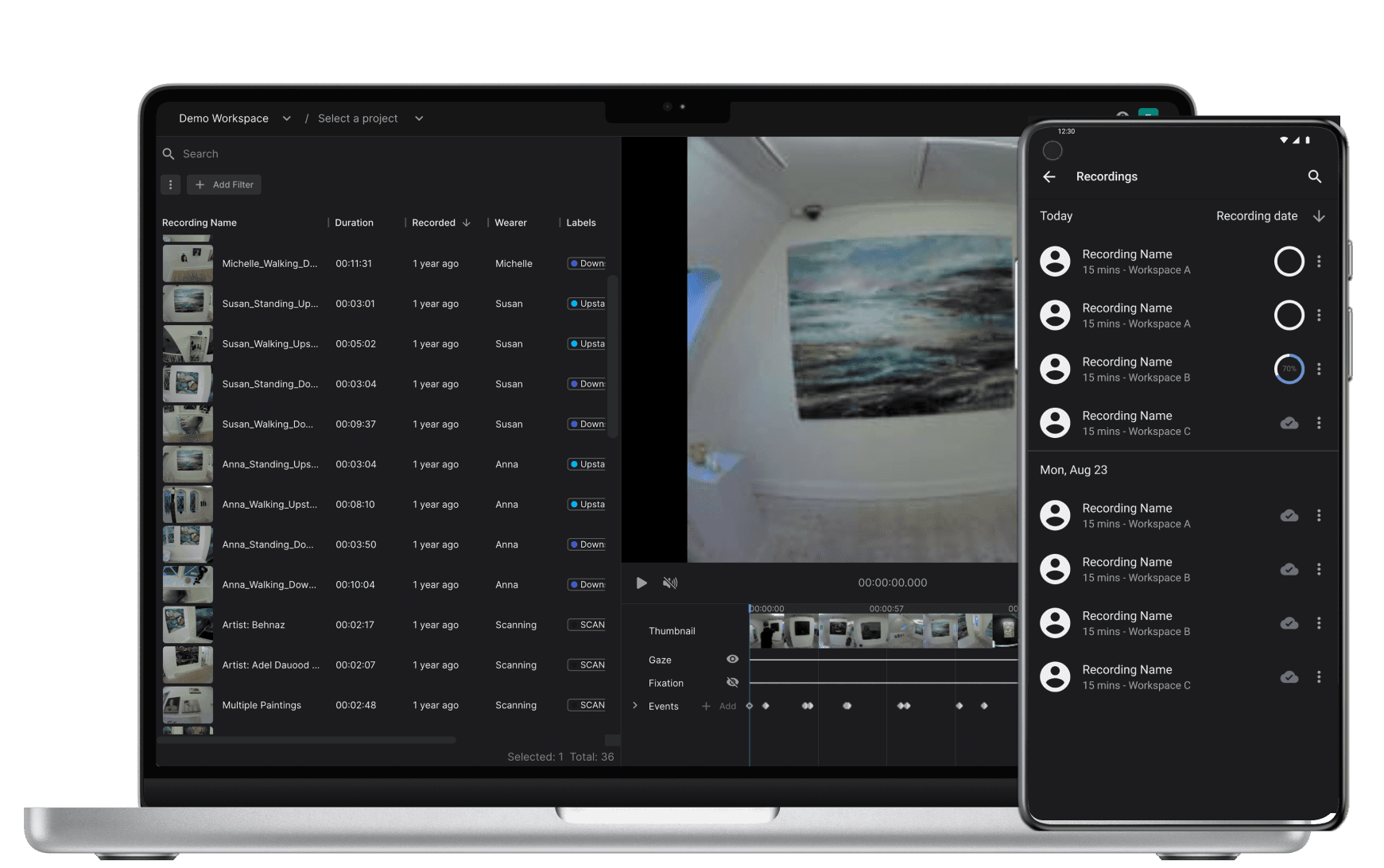In this image, a computer screen and a smartphone are positioned side by side, with the computer screen on the left and the phone on the right. The computer screen displays a detailed interface labeled "Demo Workspace," prompting the user to "Select a Project." The top portion of the screen features columns filled with various information. There's a prominent search bar for typing queries and an option to add filters.

The data presented begins with "Recording Name," followed by sections featuring numerous thumbnail images. Each thumbnail is associated with titles such as "Multiple Paintings," "Susan Standing," "Susan Walking," etc. Adjacent to these thumbnails, there's information on the duration of each recording, all timestamped as "One year ago." Further along these records, the column labeled "Wearer" lists names of different individuals, with the exception of three entries at the bottom marked as "Scanning."

Another column titled "Labels" features several entries marked with a blue dot, accompanied by labels like "Update," "Down," or "Scan" at the bottom. On the right, the smartphone screen mirrors the computer's interface showing recording names, demonstrating the synchrony between the two devices.